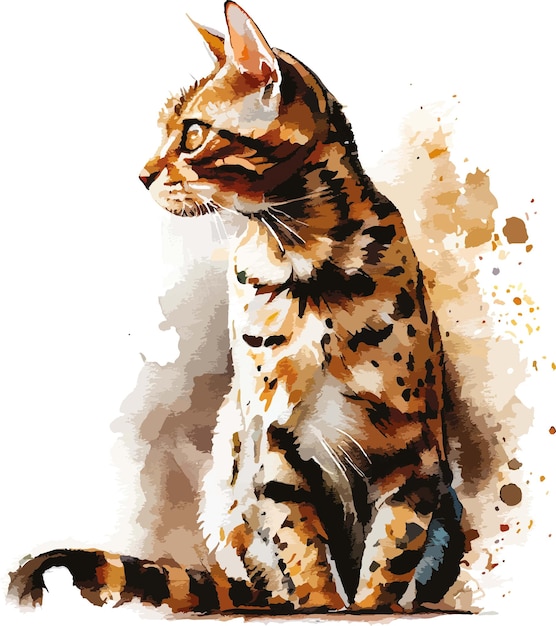The image depicts a watercolor painting of a seated cat, which appears to be a calico with a blend of light brown, orange, black, and white fur. The cat is positioned with its chest facing forward, directly at the observer, while its head is turned to its right, drawing attention to its dark yellowish-orange eye. Its ears, partially white on the insides, point straight up. The cat’s front paws rest on the ground, supporting it in its seated posture, and a tuft of white fur is visible on its belly. Notably, the left front leg is predominantly black. Its tail, striped with black and orange-ish brown, extends out to its left. The background highlights the cat against a partly visible orangey floor with a white wall adorned with splotches of different hues, including shades of brown, orange, and tan, giving an impression of paint splatters around it.